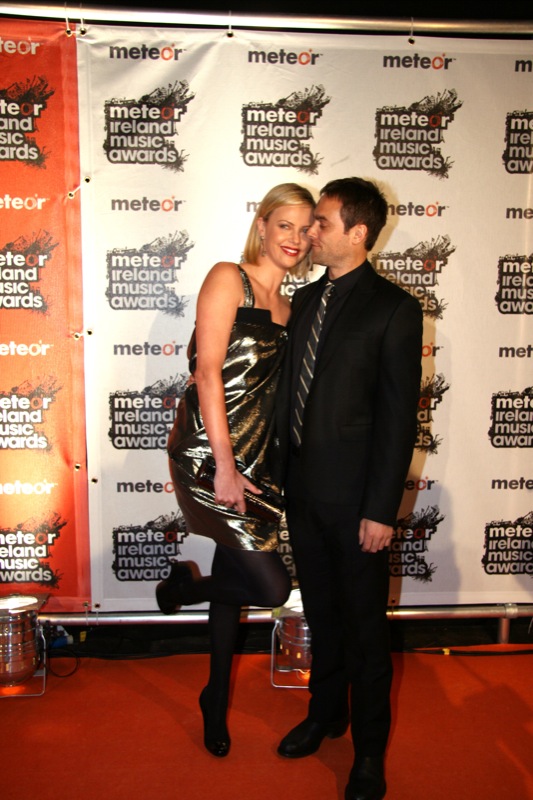In this image, a stylishly dressed woman and a man are attending the Meteor Ireland Music Awards, standing on a red carpet with a repeating backdrop of the event's logo and banners. The woman, gazing directly at the camera, is wearing a knee-length silver or grayish dress—possibly black—paired with black boots. She has one leg bent at the knee, adding a playful touch to her pose. The man beside her, dressed in a sharply tailored black suit with a black and white striped tie, appears to be leaning in for a kiss on her cheek. Behind them, a series of banners feature the event's name, "Meteor Ireland Music Awards," with the distinctive "O" in "Meteor" colored red or orange, set against contrasting backgrounds of black and white. A silver pole runs across the bottom, adorned with lights on the left side that shine up at the display. The scene captures a moment of affectionate interaction against a backdrop that highlights the prestigious event they are attending.